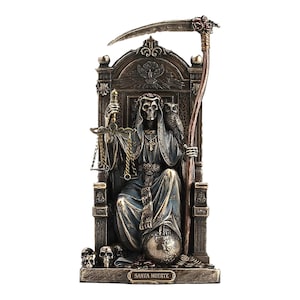The image is a color illustration in portrait orientation, depicting a highly detailed statue of the Grim Reaper, also known as Santa Muerte. The skeletal figure is seated on a tall, high-backed throne adorned with an eagle at its upper back and several skulls scattered on the floor to the left side. The Grim Reaper is wearing a long gown and a head veil, with long threads extending down towards its chest. His left foot is raised and balanced on a round silver ball, while the other foot rests on the floor. In his right hand, he holds a set of scales, symbolizing justice, and in his left hand, he wields a long bronze rod with a sharp, pointy horizontal attachment at the upper end, resembling a scythe. An owl is perched on his left shoulder, and a plaque at the base of the throne reads "Santa Muerte." The throne itself is primarily black and silver, enhancing the statue's somber and mystical appearance.